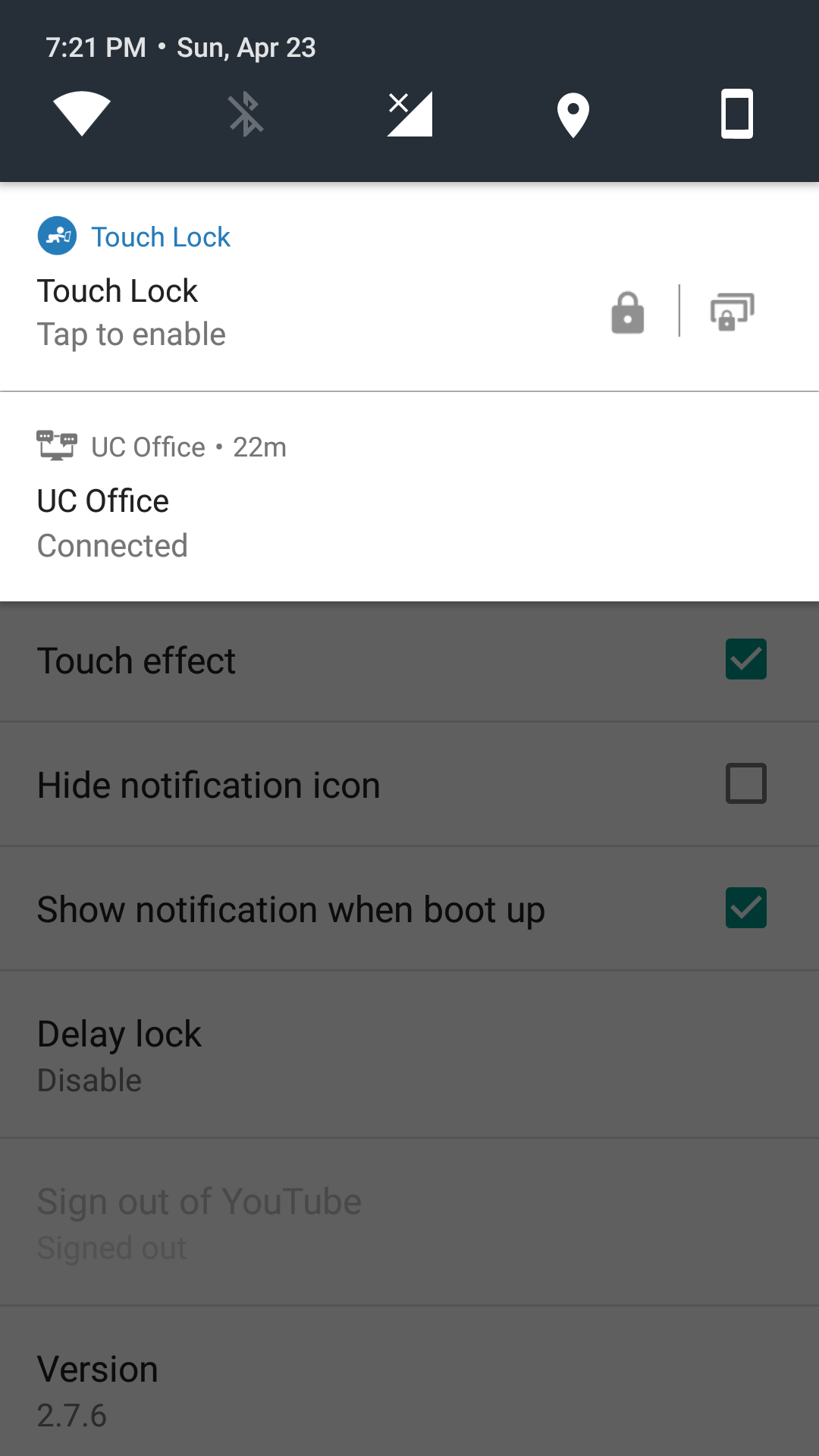Screenshot Details:

**Date and Time:**
- Timestamp: 7:21 PM, Sunday, April 23rd

**Connectivity:**
- Wi-Fi: Enabled
- Bluetooth: Disabled
- Network Signal: No bars
- Location Services: Enabled

**Screen Description:**
- The screenshot appears to be from a mobile device (either a phone or tablet).
- Background Color: White
- Text Color: Black

**Specific Sections and Features:**
1. **Touch Lock**:
   - Button Status: Locked
   - Blue Button: "Press touch lock, tap to enable"

2. **Office Connection**:
   - Status: Connected
   - Duration: 22 minutes

3. **Additional Settings**:
   - This section is grayed out
   - Options Include:
     - **Touch Effect**: Enabled (checked)
     - **Notification Icon**: Disabled (unchecked)
     - **Show Notifications on Boot Up**: Enabled (checked)
     - **Delay Lock**: Disabled
     - **Sign Out of YouTube**: Currently signed out

**App Information:**
- Version: 2.7.6

**Overall Summary:**
- The screenshot showcases someone adjusting the security settings on their mobile device. The touch lock is activated, while detailed options such as touch effect and notification display preferences are visible, indicating a customization of alert and locking behavior on the device.